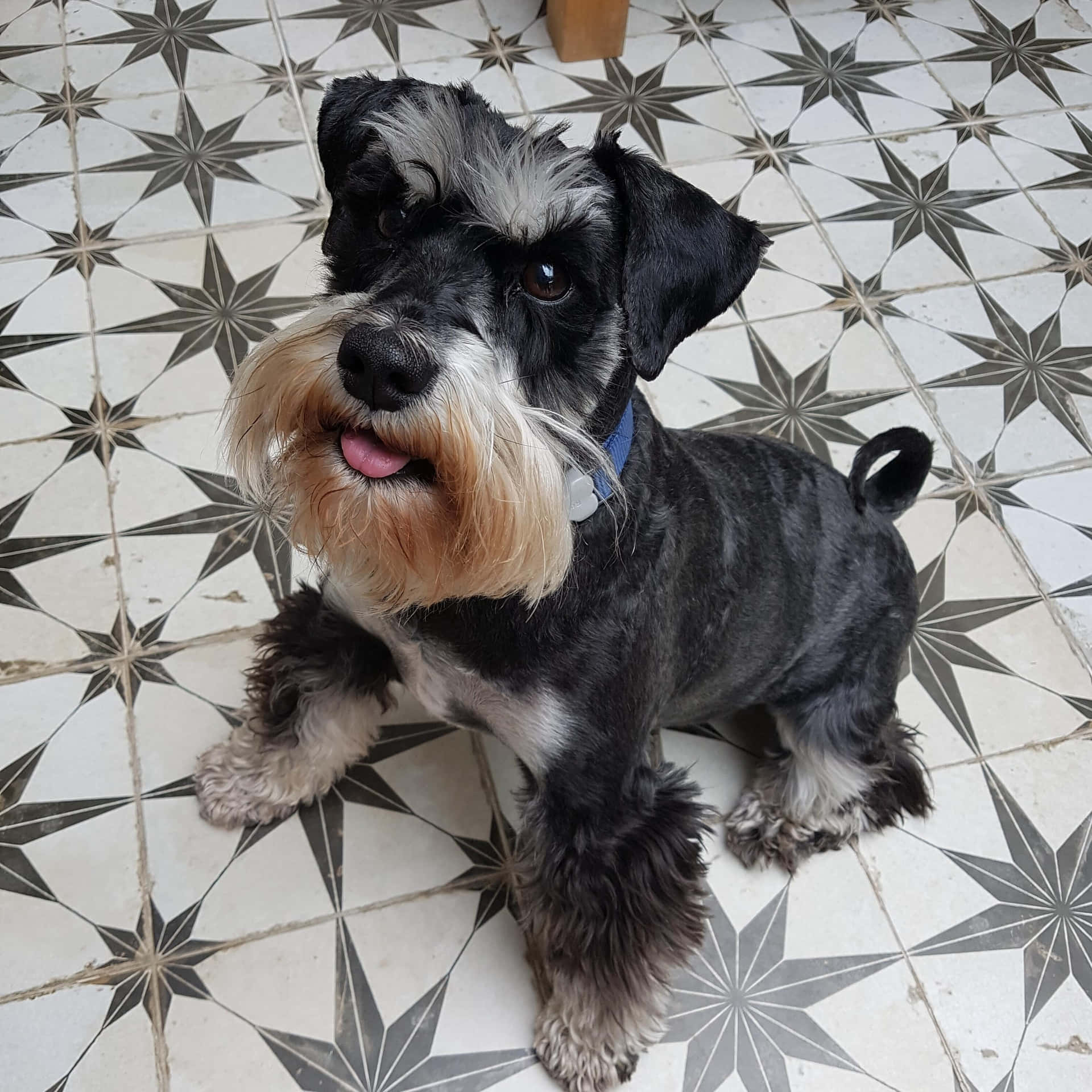The photograph captures an adorable schnauzer puppy, characterized by its predominantly black fur with distinctive white patches on its legs, chest, and the area around its mouth and nose. The dog has expressive brown eyes and a black nose, with grayish white fur over its eyes resembling eyebrows that give it a thoughtful look. The puppy's pink tongue peeks out slightly, contributing to an appearance that almost seems like it's smiling. A blue collar with a gray clasp adorns its neck. The dog is standing on a white tiled floor featuring a pattern of black and gray stars, some of which show signs of dirt. The puppy’s fur varies in length, with longer fur on its legs and a shorter coat covering the rest of its body, suggesting a recent grooming. The small tail is slightly curled, enhancing its playful demeanor. The dog looks up eagerly at the person taking the photograph, as if anticipating a treat or a walk.